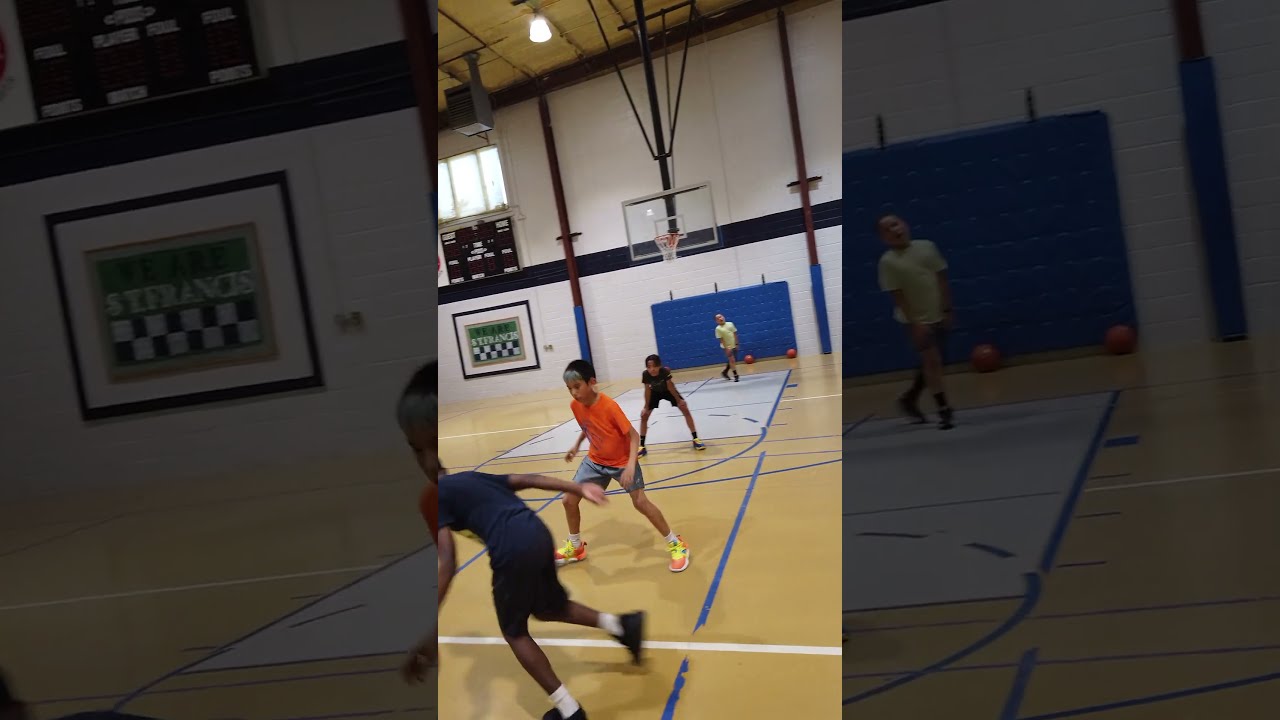The photograph captures an indoor gymnasium, intricately divided into three panels with differing light levels. The center panel is brightly lit, showcasing a moment on a standard beige-colored basketball court furnished with white and blue lines. Under a ceiling light, four adolescents—likely aged between 13 and 15—engage in a casual basketball game. From left to right: one player, partially cropped out, runs towards the left; another in an orange shirt stands with legs apart; a third player stands similarly with hands on knees; and the fourth wearing a yellow shirt loiters near the basketball hoop. The walls are adorned with a plaque reading "St. Francis" and a scoreboard displaying “foul player” with no numerical data. The left and right dark-shaded panels are blown-up sections from the central image, with the right including a blue cushion on the wall. Together, these panels provide a detailed and layered depiction of the scene.